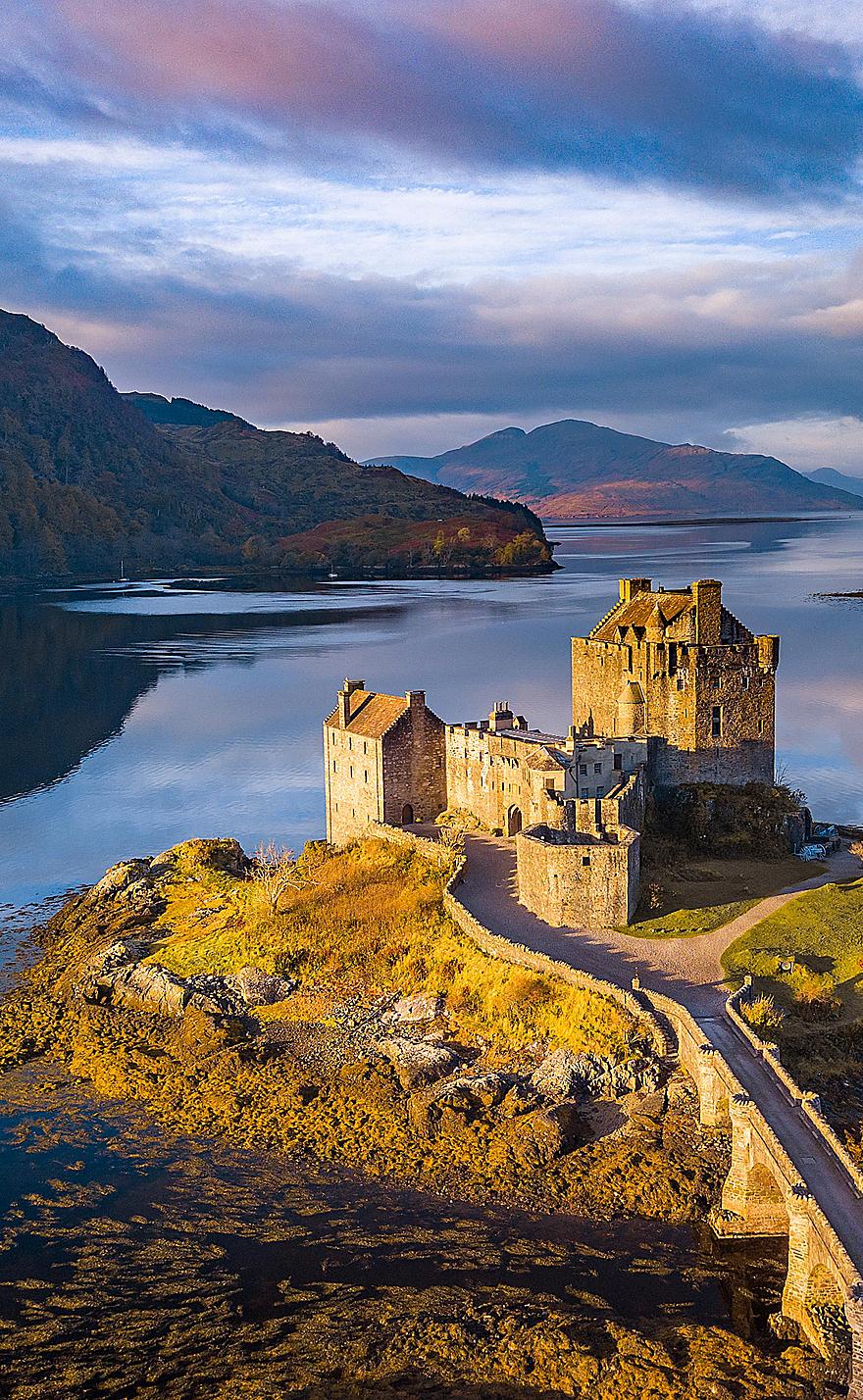Captured from an aerial perspective, this enchanting image showcases a majestic, ancient castle situated on a tiny, verdant island, surrounded by dark, mossy waters. The castle, rendered in white, gray, and brown stones, boasts a reddish, chimney-studded roof and comprises multiple interconnected buildings, including a distinctive tall, triangular structure and a smaller, rectangular edifice. A stone arch bridge with a pathway of brown bricks extends from the lower right of the image, providing access to the castle, with a lengthy gravel driveway leading to the complex. The landscape around the castle is lush with greenery, punctuated by the detailed stone steps and pathways.

In the background, the serene lake is framed by jagged, brown mountains, and the sky above is layered with dramatic hues of dark blue, light purple, and light blue swirled with white clouds. The distant right-hand corner of the image reveals a mountain cloaked in trees, harmonizing with another tree-adorned hill on the left, encapsulating the timeless beauty of this historic sanctuary.